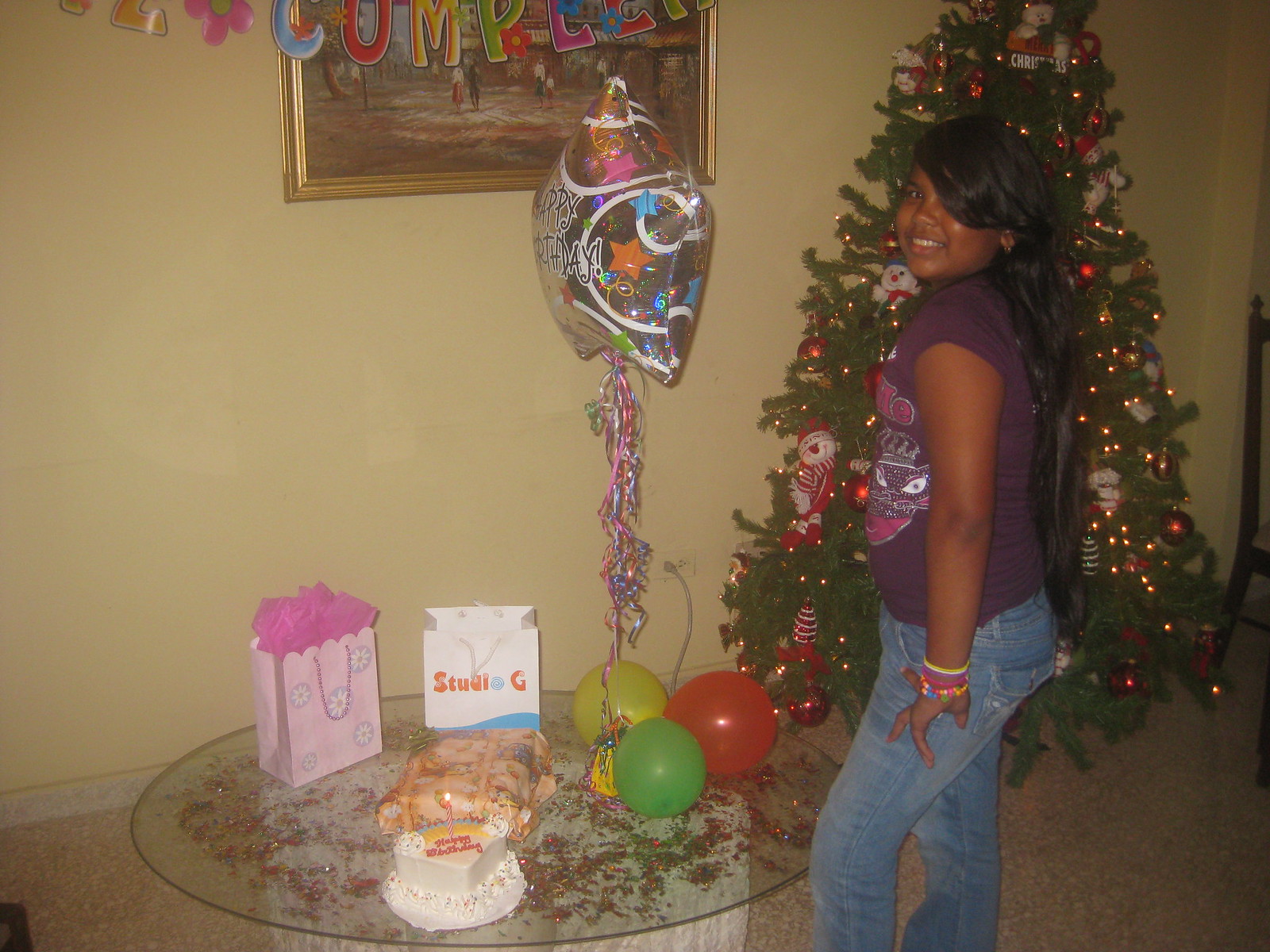In the image, a young, dark-skinned girl with a radiant smile stands in the last third of the picture, posing in front of a festive Christmas tree, suggesting the holiday season. Her long black hair, styled possibly with a weave, drapes over one eye, accentuating her youthful charm. She wears a purple t-shirt adorned with a design, possibly a cat with a crown, and blue dungarees. Accessorizing her outfit, she has fabric-like bracelets on her wrist.

To her left, a circular table is laden with colorful presents, a birthday cake, and a variety of balloons, including a large 'Happy Birthday' balloon, hinting that her birthday coincides with the festive season. The setting is an indoor, carpeted room with a tan, yellowish wall in the background, featuring a framed painting partially obscured by a banner. The area is vibrant with the colors pink, green, blue, red, yellow, gray, silver, clear, purple, and orange, creating a lively, celebratory atmosphere.